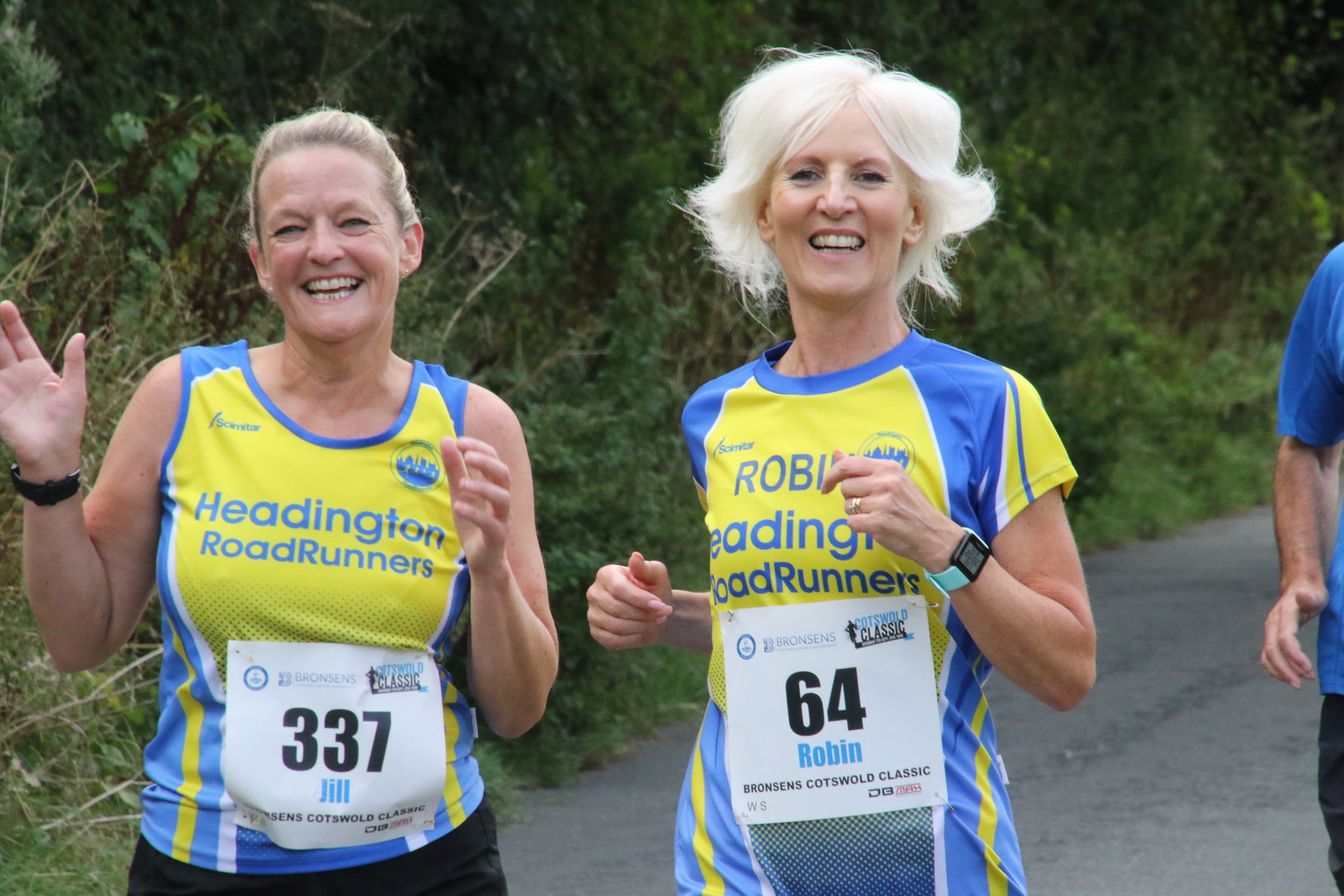This vibrant photo captures two older women running enthusiastically in a race, likely a marathon. Both women are smiling, radiating joy and camaraderie. On the left, a slightly younger-looking woman with either short or tied-back hair wearing a blue and yellow nylon tank top and showing plaque number 337 labeled "Jill." On the right, the other woman, with flowy blonde hair, dons a matching blue and yellow t-shirt, marked with plaque number 64 labeled "Robin." The shirts bear the inscription "Headington Roadrunners." They appear to be running on a concrete or street path, surrounded by lush green trees and shrubbery, indicating a beautiful, natural setting. Despite their age, they exude vitality and happiness as they participate in this event together.